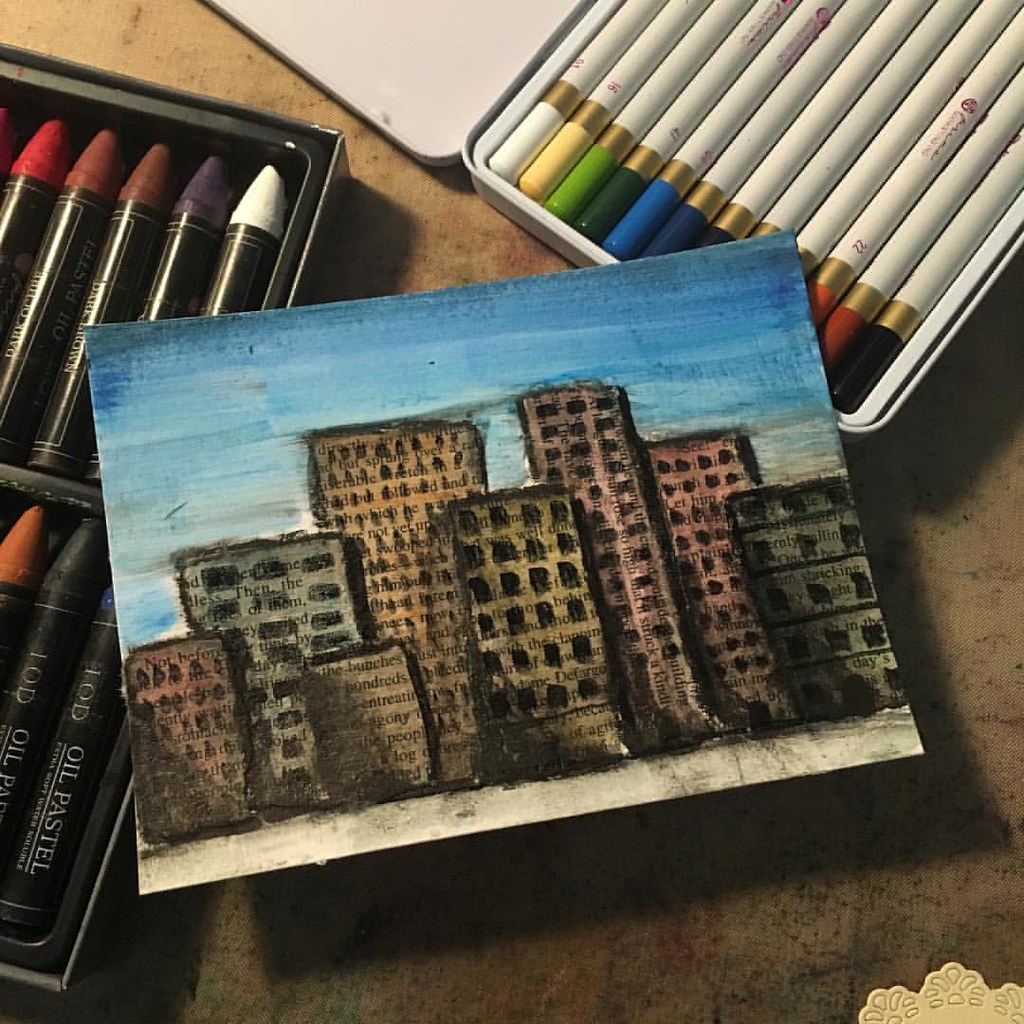This image is an up-close photograph looking down at a piece of art on a table. The artwork is a small piece of paper featuring a cityscape with multiple colorful buildings. The buildings are of various hues, including green, orange, red, and are heavily outlined in black. They appear to be many stories tall and have black windows. The sky above the buildings is a smudgy blue, resembling a watercolor wash. Interestingly, the buildings are constructed with cut-out pieces of newsprint, pasted into rectangular shapes, and overlaid with oil pastels and colored pencils. The paper on which the drawing is done shows some white spaces with a few stains.

The artwork is laid atop a metal container of colored pencils on the right side, while a container of oil pastels is on the left. The colored pencils, housed in a white metal tin, are indicated by their colored tips in shades of white, yellow, green, dark green, light blue, dark blue, black, and red. The oil pastels, in a black plastic container, are predominantly in browns, but also include reds, blacks, and a bright white pastel. 

This entire setup rests on a brown and red colored table, possibly made of stone or granite. Additionally, at the very lower right-hand corner of the image, there is a small doily with rippled edges, resembling a flower, barely visible in the photograph.